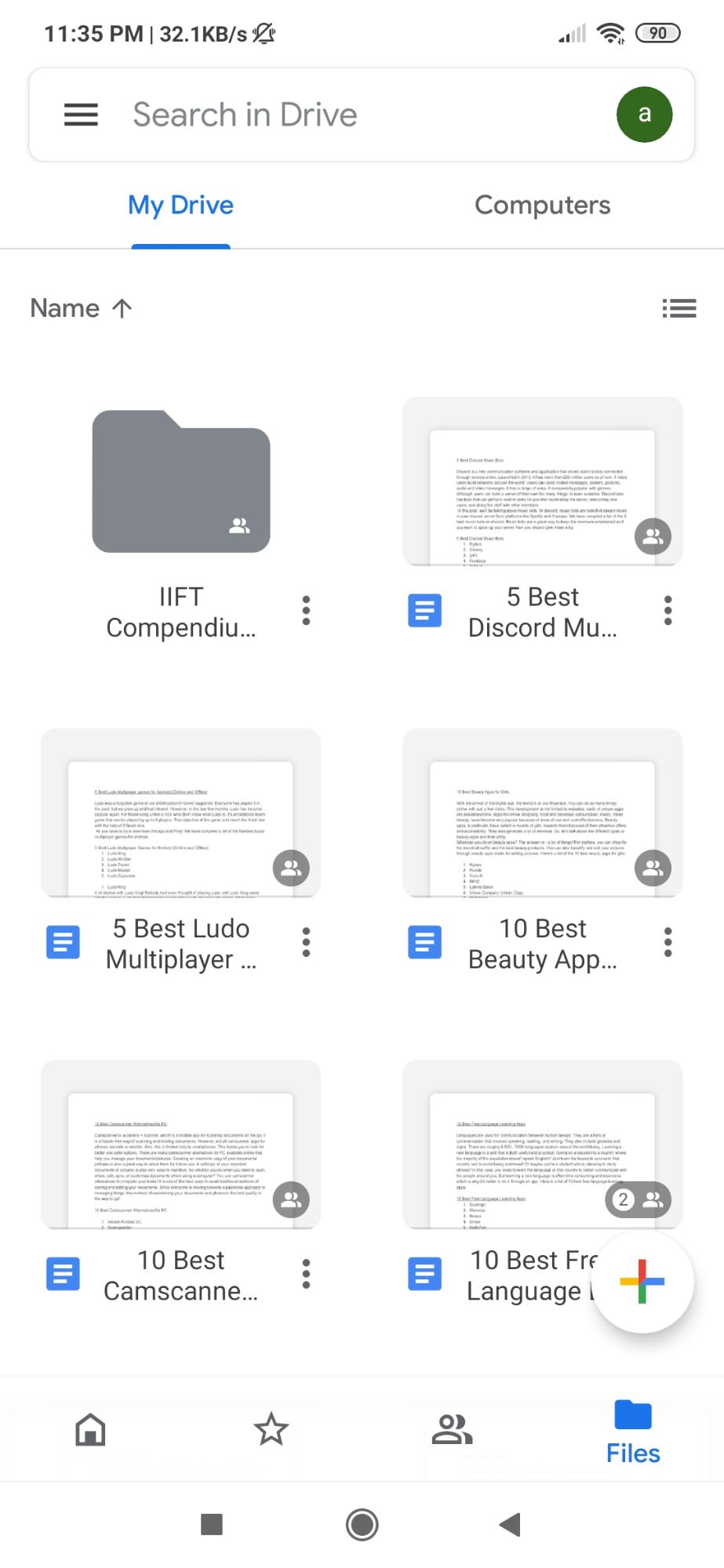This image, captured from a cell phone, shows a screen with various details at a glance. The device has a battery life of 90% and a strong connection, and the time displayed is 11:35. At the top of the screen is a white search bar featuring three horizontal lines on the left, indicating a menu option. The text inside the search bar reads "Search in Drive," and there is a large black circle with an "A" symbol.

Beneath the search bar, there are menu options labeled "My Drive" and "Computers," with "My Drive" highlighted in blue and underlined with a blue bar. The next section lists file names and their details. The list starts with a file named "IIFT can bend you," represented by a dark black page. Following that are several files with gray borders and extensive writing:

1. "Five best Discord MU" - an image with a light gray background and a lot of text.
2. "Five best Ludo multiplayer" - similar in style with a gray border and text.
3. "10-bit app" - another file with a gray border and text.
4. "10 best" followed by "Cam scanned" - again, a gray border and text.
5. "10 best something language" - partially obscured by a white circle with a Google Plus sign.

Each file entry has a gray circle icon next to it, with the last one having a '2' inside a white circle within the gray circle.

At the bottom of the screen, "Your files" is highlighted in blue, indicating that these are the files currently displayed. The bottom navigation includes icons such as a home button, a star, and a person image. The lower portion of the screen shows a home button, a black box on the left, and an arrow pointing left on the right.